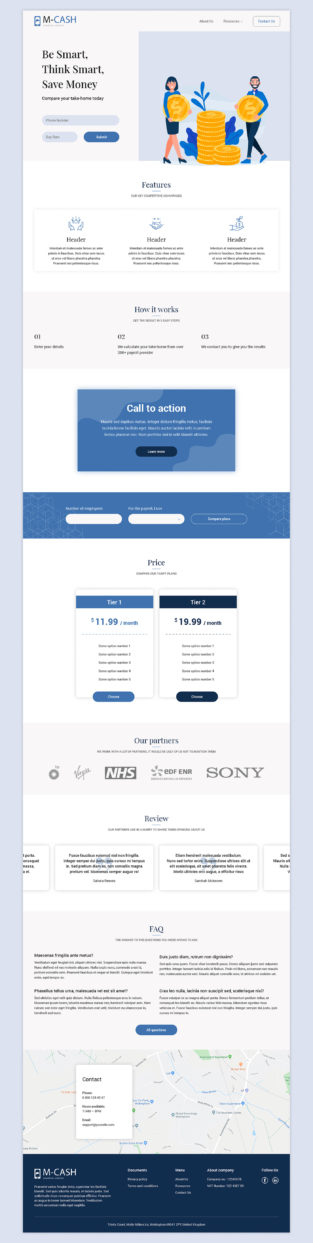This image captures the landing page of a website named "M-Cache." The page features a light blue background with a central white vertical rectangular box containing various elements including icons, images, and text. While much of the text is too small to read, the top section stands out with an image set against a light blue background. This image depicts a man on the right and a woman on the left, both smiling and holding gold coins adorned with dollar signs. Positioned next to this image, the title "Be Smart, Think Smart, Save Money" is prominently displayed. Below this title lies an abundance of additional information.

A dark blue horizontal rectangular box stands out with the call-to-action text displayed in white. Further down, pricing information is presented with two distinct boxes: one stating "$11.99" and the other "$19.99." The section labeled "Our Partners" follows, listing several partner companies, with legible names including Sony and NHS.